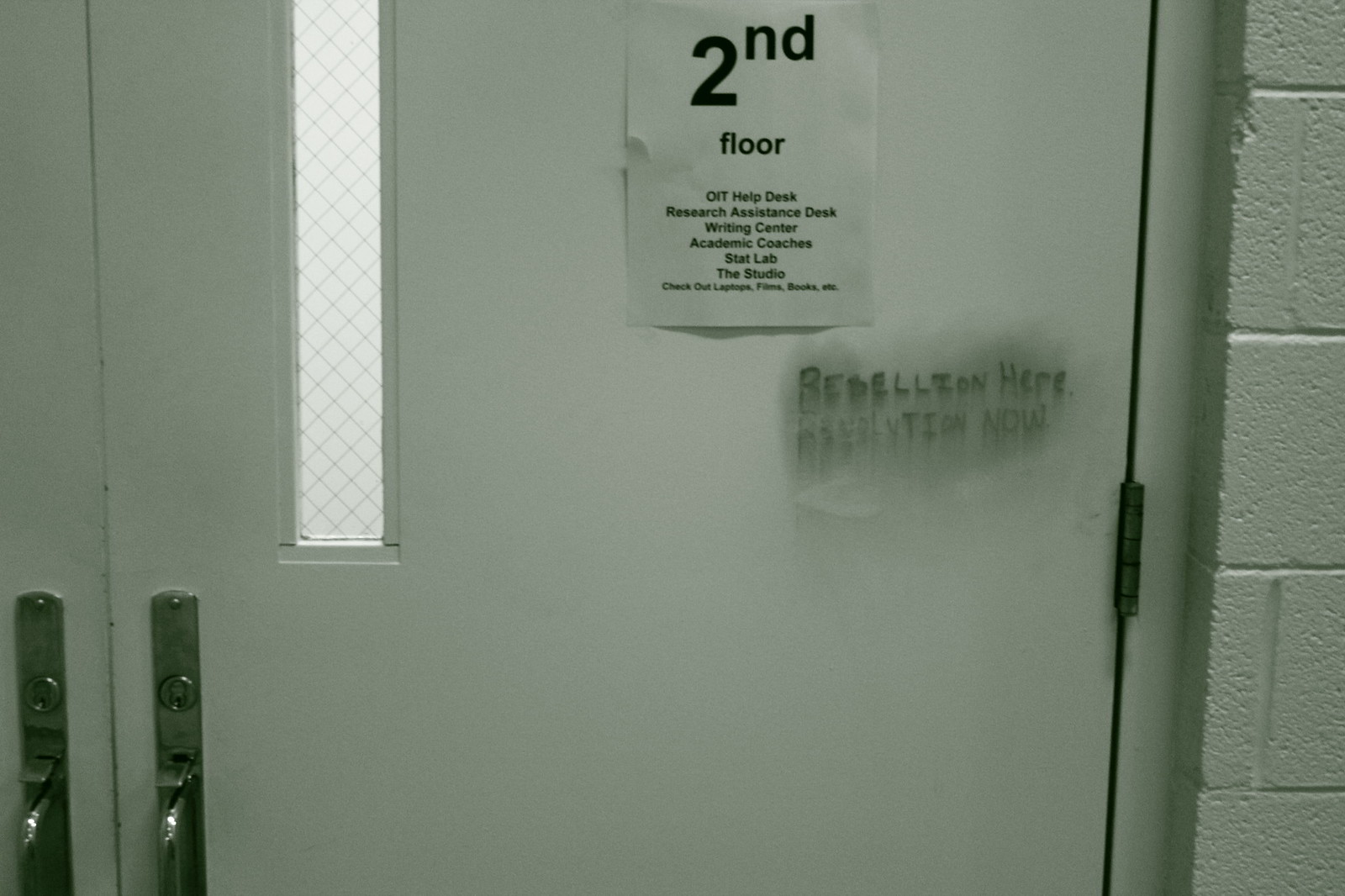The photograph captures the interior of what appears to be a cinder block building, suggesting it might be a school, jail, or similar institutional facility. Dominating the image are two doors set within the cinder block wall. Both doors feature pull handles, enabling them to be opened manually. The door on the right bears a sign indicating the amenities located on the second floor. The top line reads "Second Floor," with text beneath listing "Writing Center" and "Lab," hinting strongly at an educational setting such as a school. Additional text is present but illegible, although the impression of a list of facilities is conveyed. Beneath the printed text, there's a patch of handwritten graffiti—some partially erased words, possibly containing unpleasant content, are still faintly visible, adding a touch of rebellion or casual disregard to the otherwise institutional atmosphere.